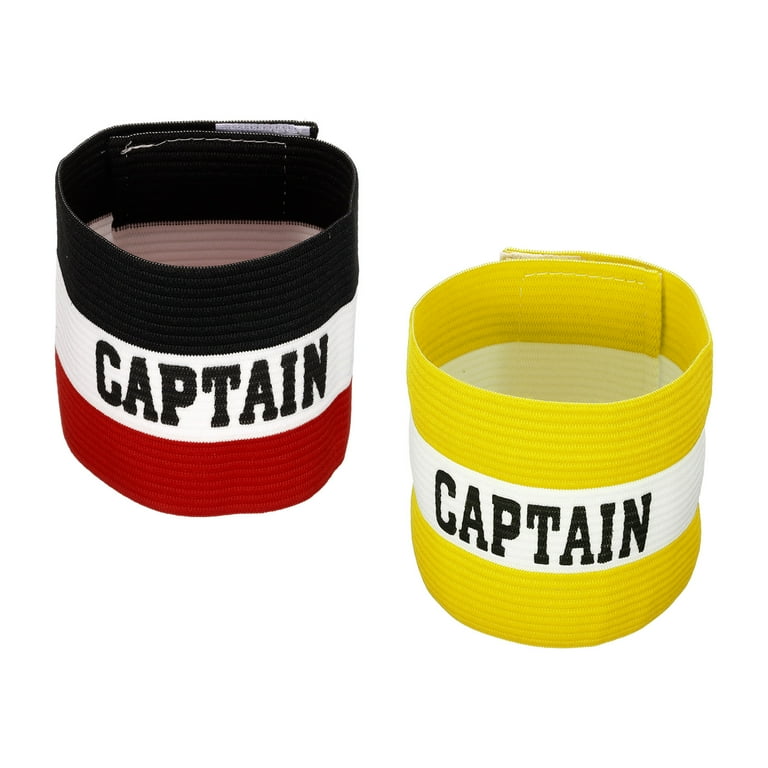This close-up image showcases two armbands designed for sporting events such as football or rowing. Both armbands are cylindrical in shape and secured with white Velcro straps. The armband on the left features a bold, tri-color design with horizontal stripes in black, white, and red. The white center stripe prominently displays the word "CAPTAIN" in black, capital letters, written in a serif font. The armband on the right is primarily yellow, with a white center stripe that also bears the word "CAPTAIN" in the same black, capital letters. The textured, cloth-like material of both armbands includes rivets, adding depth to their appearance. In the image, the yellow armband appears slightly closer to the viewer, while the red, white, and black armband is set slightly farther back. Both items are presented side by side, albeit slightly askew, emphasizing their roles as captain's identifiers in different sports contexts.